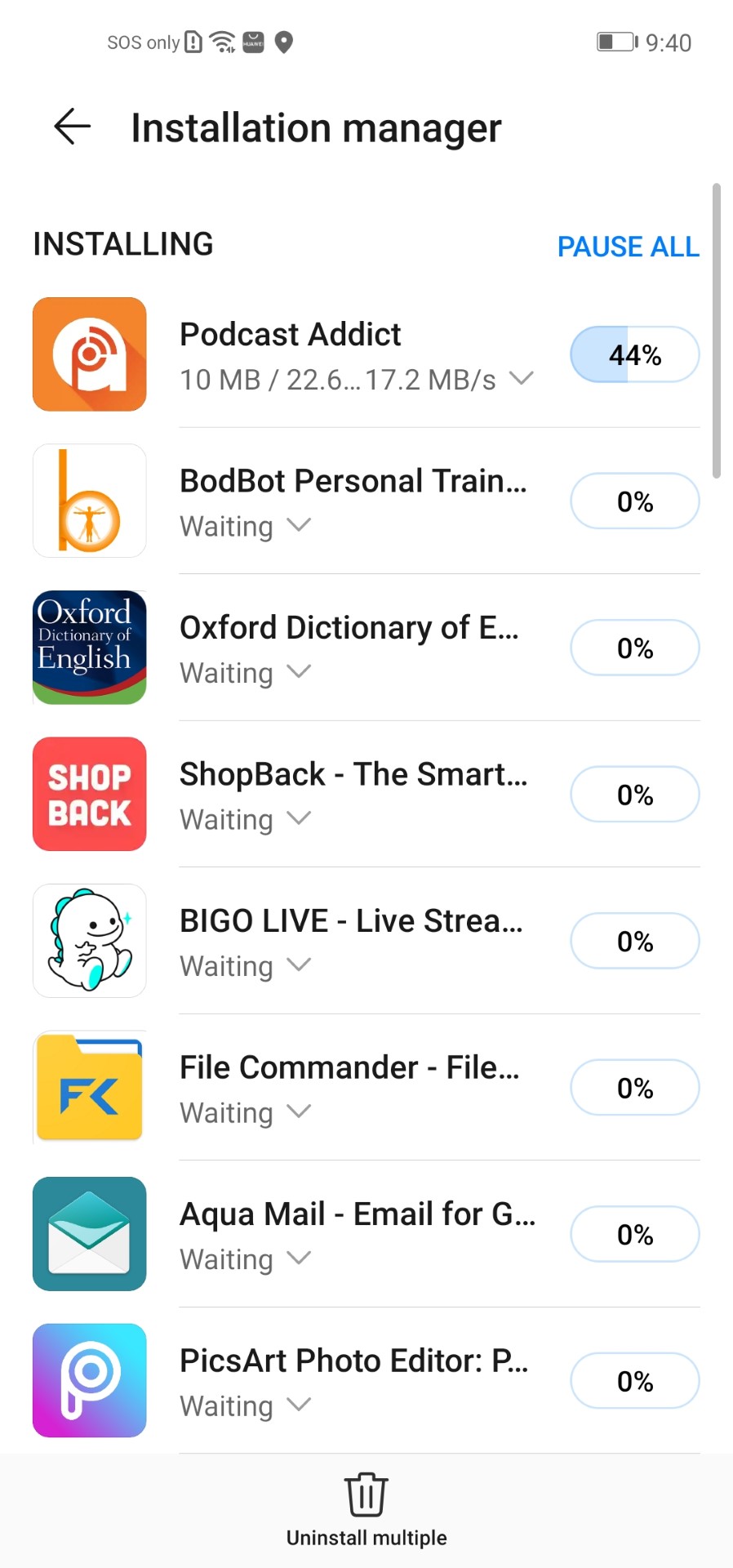The image appears to be a screenshot of a smartphone screen. At the very top, the notification bar displays common symbols: the Wi-Fi icon, battery charging indicator, and the current time, 9:40 AM. An arrow icon pointing left signifies navigation, while the text "Installation Manager" is prominently displayed. Below this, the screen shows a list of several apps currently being installed:

1. Podcast Addict (orange icon)
2. BodBot Personal Training (blue icon)
3. Oxford Dictionary of English (red icon)
4. ShopBack (green icon)
5. BIGO LIVE - Live Streaming (pink icon)
6. File Commander (yellow icon)
7. Aqua Mail (teal icon)
8. PicsArt (purple icon)

On the top right-hand side, the option "Pause All" is written in blue letters. Each app listed is accompanied by its respective colorful icon. At the bottom of this list, a trash can icon is visible with the text "Uninstall Multiple," offering the option to remove several apps at once. The vibrant variety of app icons adds a colorful touch to the interface.